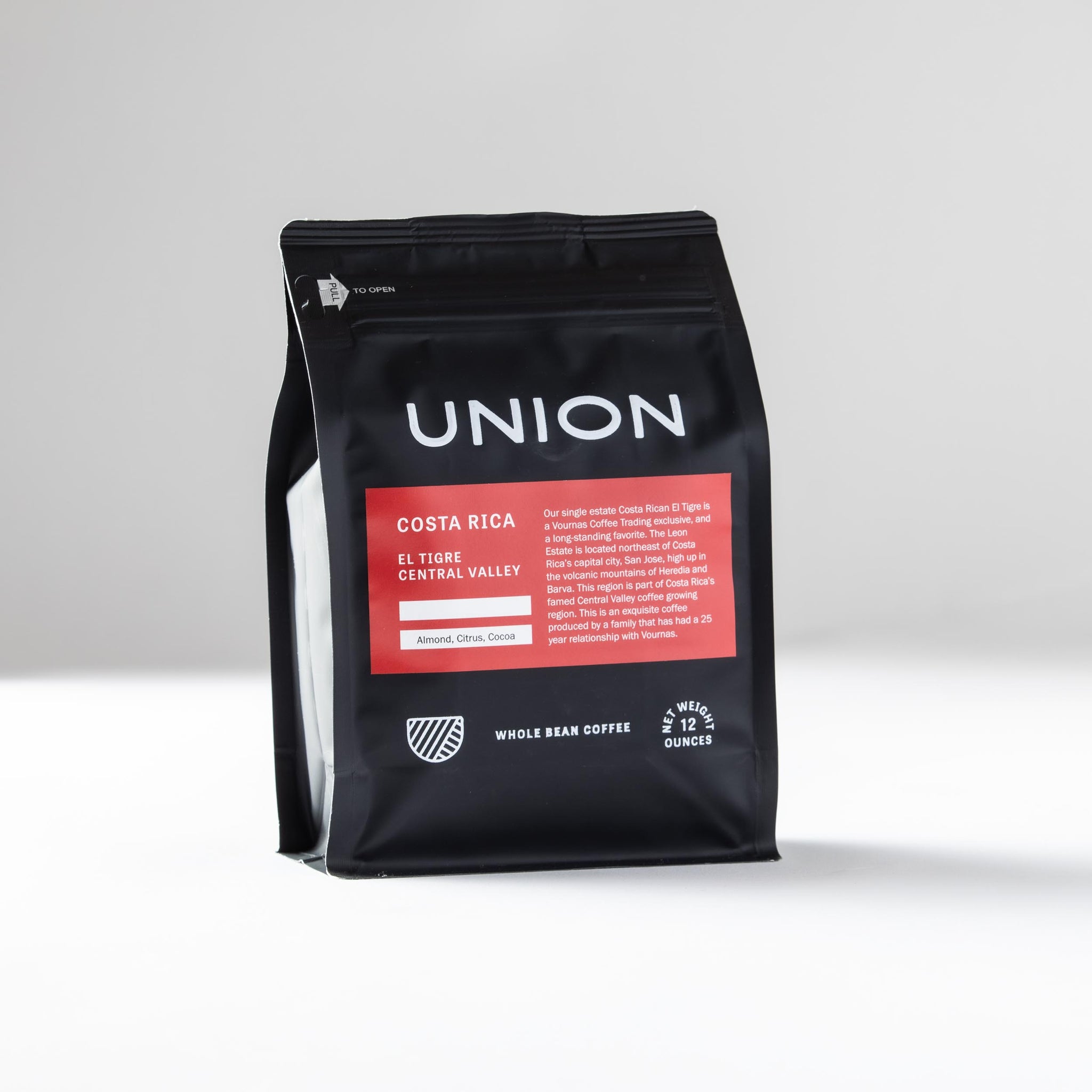The image depicts a small, sealed black bag of whole bean coffee from the Union brand. The brand name "Union" is prominently displayed in white text at the top of the bag, while at the bottom, it states "Whole Bean Coffee" and "Net Weight 12 ounces". A red rectangular label in the center features white text reading "Costa Rica El Tigre Central Valley" along with flavor notes such as almond, citrus, and cocoa. Additionally, a paragraph on the left side of the rectangle provides detailed information, noting that the coffee is a single-estate Costa Rican variety exclusive to Verna's Coffee Trading and is described as a long-standing favorite. The photograph is set against a white and blue background.